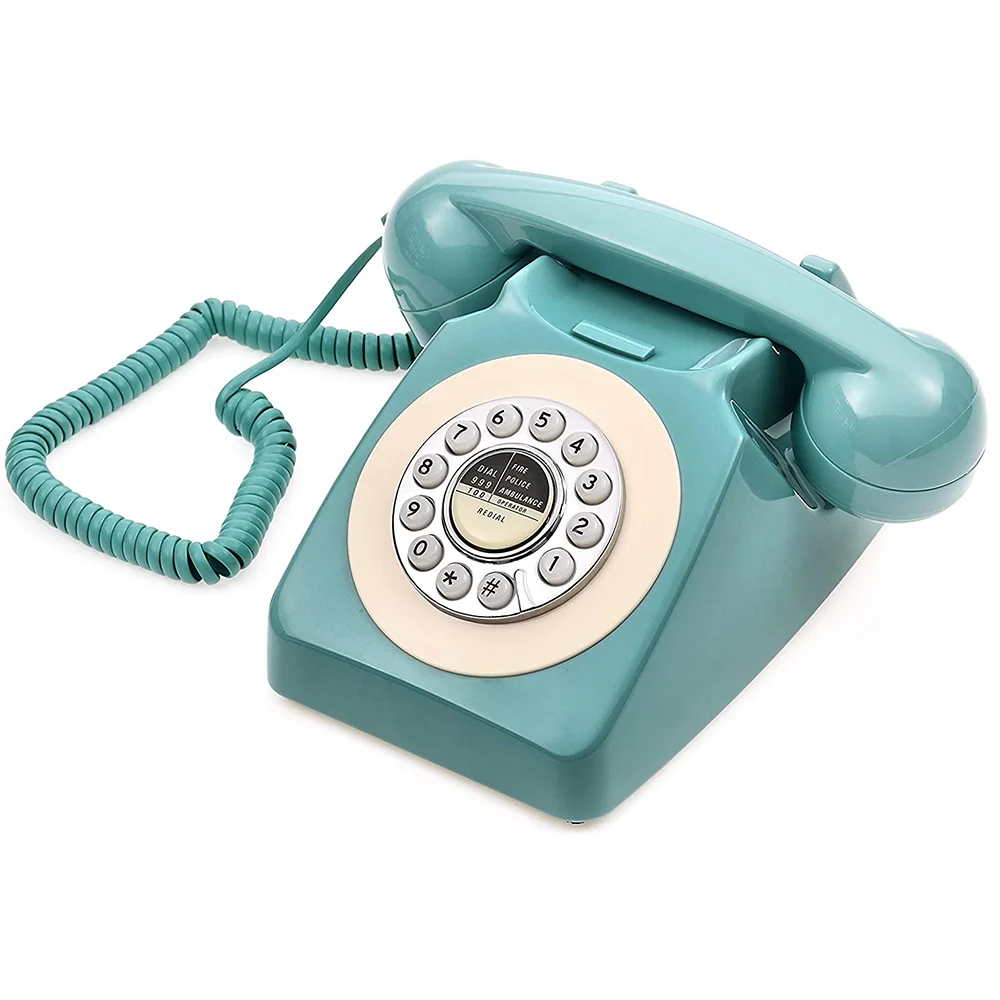This is a photograph of a vintage turquoise-colored home telephone with a glossy finish, captured against a white background. The phone features a corded, spiral handset resting on its base, with the cord positioned to the left. The face of the phone is round and silver, housing push-button numbers from 1 to 0, along with star and pound symbols, all inscribed in black on white buttons. The phone's center dial area displays essential emergency contact instructions—such as Fire, Police, Ambulance (Dial 999 or 100), Operator, and Redial—highlighted in black text. The overall retro design evokes a classic feel, reminiscent of older telephones that plugged into the wall.